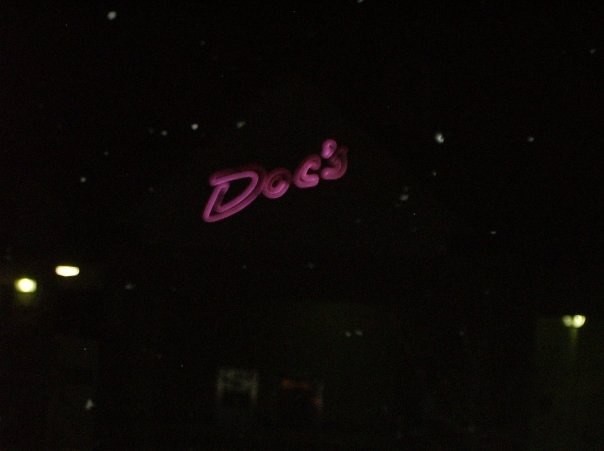In the photograph, taken in a dimly lit setting, it is nearly impossible to discern whether the location is indoors or outdoors. The scene might depict an enclosed theater or perhaps an open-air theater shrouded in darkness. On the left side of the image, a couple of faint lights are noticeable, while a single light on the right side suggests either outdoor or indoor illumination. Central to the composition is what appears to be a screen, although the obscurity makes this uncertain. The screen, seemingly in the middle of the frame, displays the word "DOCS" in a pink, plastic-like or clay-like font. Surrounding this text are elements resembling stars, but the overall blurriness renders precise identification difficult.